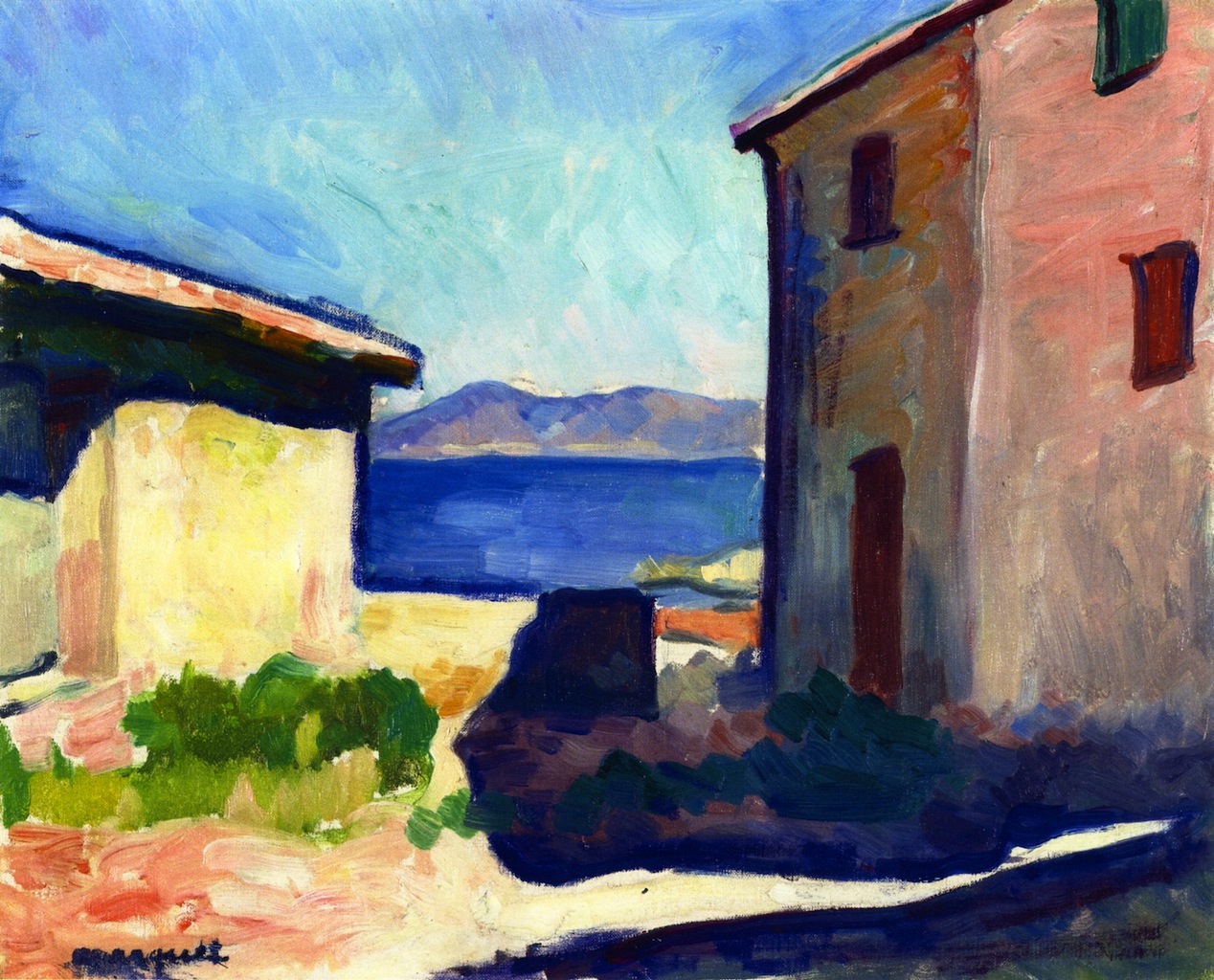This colorful, post-impressionist watercolor painting titled "House at Saint-Tropez" by Albert Marquet, created in 1905, vividly captures a landscape scene in a hot, dry climate with minimalist yet striking details. In the foreground, there are two partially visible houses: the house on the right is a two-story pink stucco with red windows and doors, while the house on the left is a shorter yellow stucco building with a red tile roof. These homes are separated by a grassy courtyard adorned with green plants and bordered by red dirt. A dark road winds around the yellow house, leading towards a distant, serene blue body of water, possibly a lake or ocean. Beyond the water lies a rugged range of brown mountains under a blue sky tinged with white. The painting uses a palette of white, various blues, purples, oranges, reds, browns, tans, and greens, bringing a vibrant, yet tranquil feel to this scene devoid of people or animals.